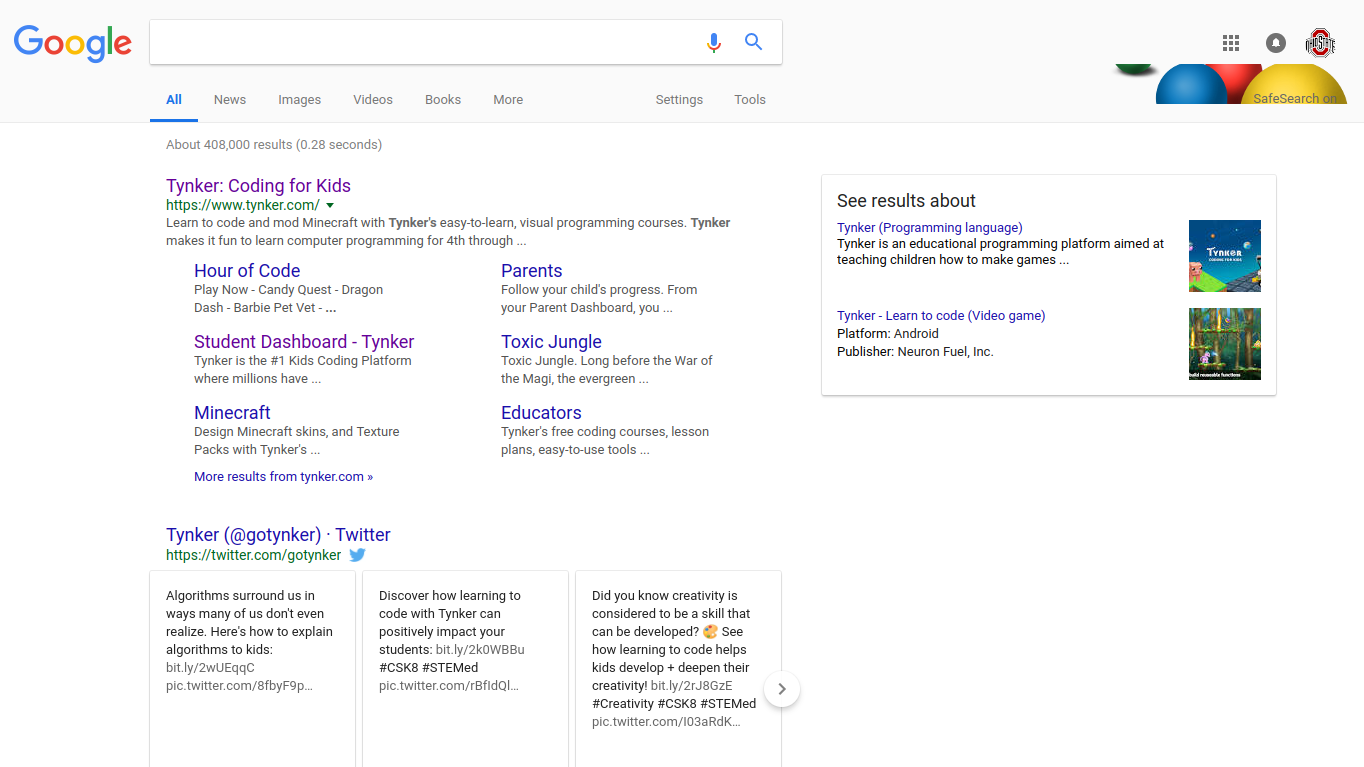The image depicts a Google search results page. The classic Google logo sits prominently at the top left, with the search box placed just below it—currently, it's empty. Beneath the search bar, a selection of options is visible, including: All, News, Images, Videos, Books, and More, followed by Settings and Tools.

On the right side of the page, a portion of a series of colorful 3D balls is visible. These balls, displayed in green, blue, red, and yellow, suggest some form of interactive or visual content related to safe search settings. Above them, there is a small round icon featuring a red and white mascot with some black writing, though the details are not entirely discernible even when zoomed in closely.

The first search result showcases "Tynker: Coding for Kids" from the URL tynker.com, advertising various educational tools such as the Hour of Code, parent and student dashboards, and coding platforms like Tynker Toxic Jungle and Minecraft for educators. To the right, a box provides additional context for Tynker, featuring a small blue square with what appears to be a cartoon image of a kid, resembling a keyboard and cartoon characters.

Further details reveal that Tynker is an educational program platform that helps children learn coding by creating video games. The image accompanying this information depicts a jungle or forest setting with cartoon characters, emphasizing the platform's interactive and playful approach to learning.

The subsequent result is a Twitter link to @gotynker, showing a few tweets related to the Tynker platform. However, the content of these tweets remains unread due to time constraints.